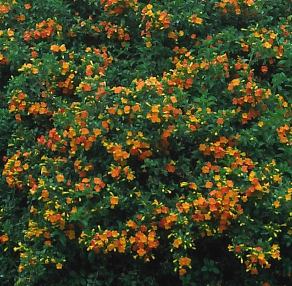This square, full-color photograph, taken outdoors during the daytime under natural light but with a dull and muted tone, captures a top-down view of a dense patch of orange flowers interspersed with dark green leaves. The image has a soft, understated aesthetic due to the overcast sky adding to the lack of significant lighting or shadows. The flowers, predominantly small and orange with a few yellowish ones, are clustered more densely in the center of the frame, while the edges, particularly at the bottom, reveal patches of dark soil beneath the leaves. The uniform, dark green foliage forms a consistent backdrop to the varied but subtle blooms, creating a calm and somewhat somber botanical scene without any animals, humans, or added text.